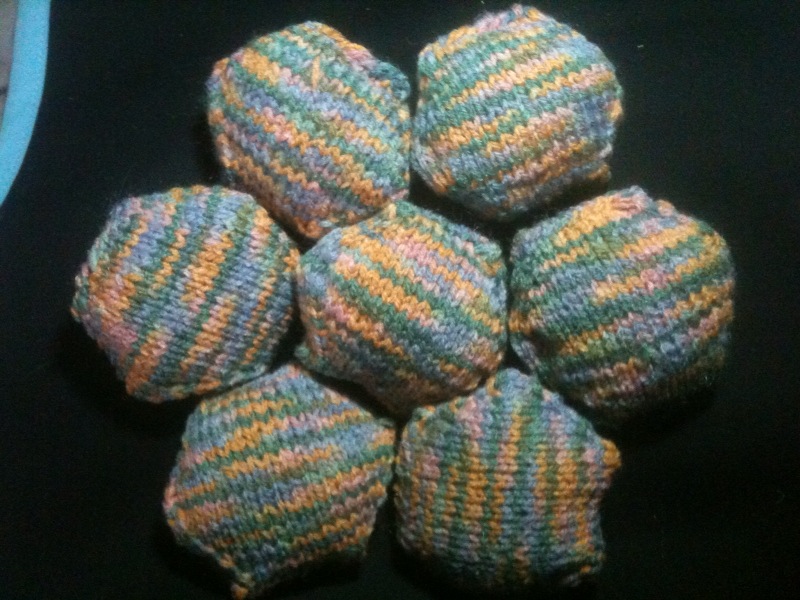The image features a simple yet intricate flower shape composed entirely of seven knitted balls, each formed from variegated yarn. All balls, including the one at the center and the six surrounding it, share the same color palette, which consists of goldenrod yellow, light pink, blue, and dark bluish-green, in an irregular pattern of stripes and patches. The balls are roughly hexagonal, three-dimensional, and are likely stuffed with some sort of filler to highlight their shape. Each ball's variegated yarn stripes run in different directions, adding to the visual complexity. This knitted flower occupies about 70% of the image and is positioned against a dark background that showcases a cloth-like texture, with a thin line of light blue stitching visible in the upper left-hand corner. Across the ensemble, the colors blend subtly, presenting a somewhat muted, pastel-like palette.